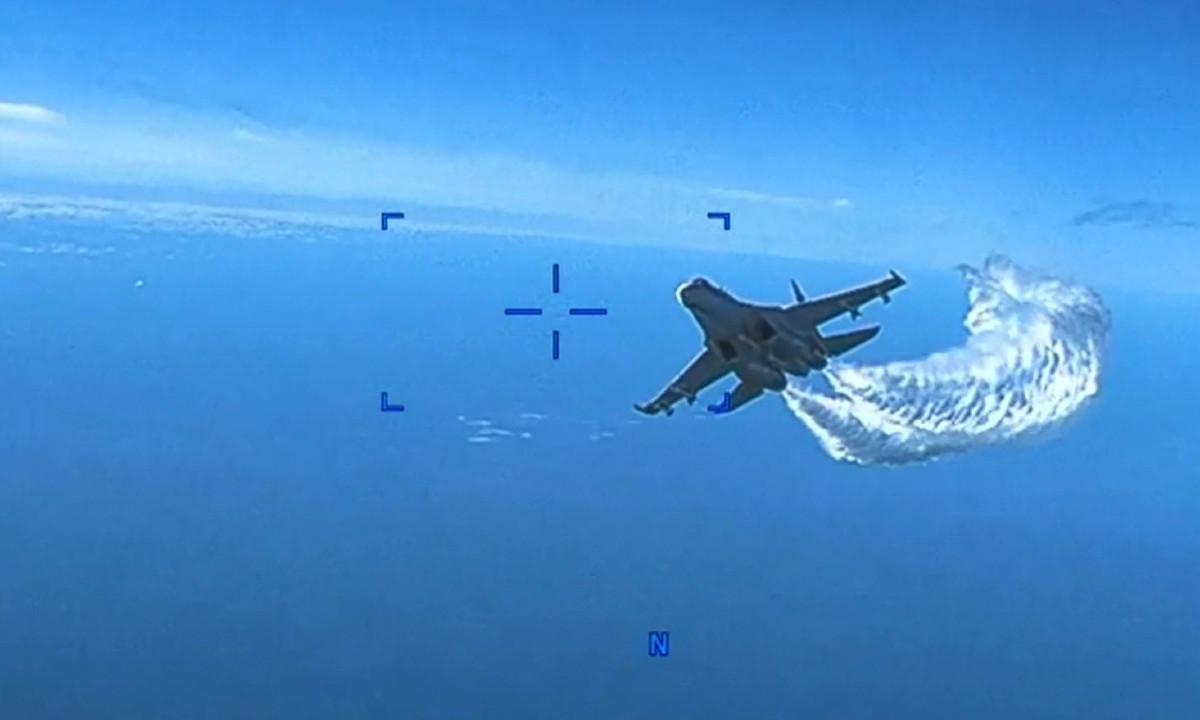The image displays a somewhat blurry close-up of a silver fighter jet accelerating in the sky. White smoke billows from its exhaust, indicating rapid movement. The jet appears to be flying over a vast body of water, possibly the ocean, with the blue horizon visible in the background. The sky shares the same blue hue as the ocean and is dotted with misty clouds, most prominently on the left side. Patches of clouds also appear near the jet. The image is framed by blue corner lines, creating a square border akin to a viewfinder, with a reticle or aim cursor centered and slightly to the left of the jet. Notably, a blue letter "N" is visible at the bottom middle of the image.